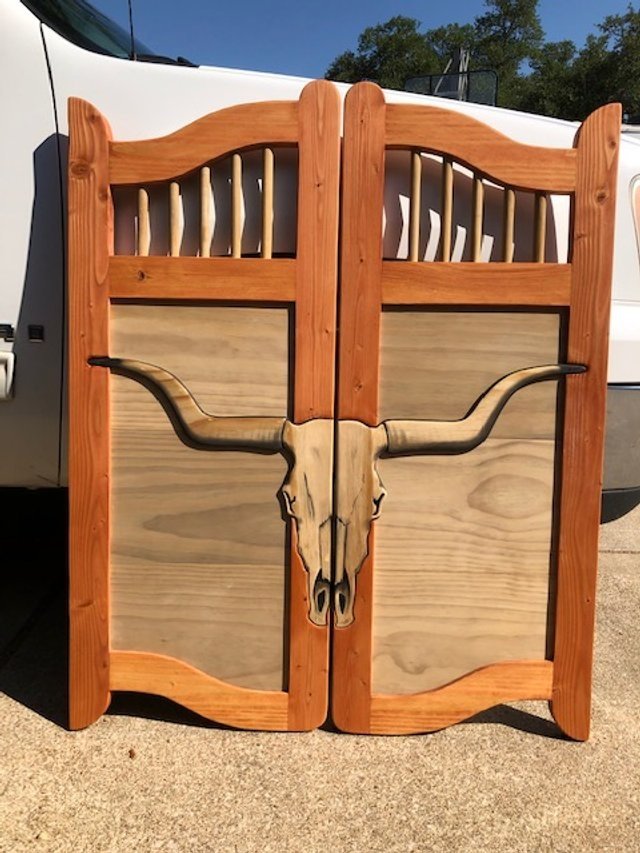This photograph, in portrait layout, captures an outdoor scene with a vibrant blue sky and distant green trees. Prominently featured in the image are handcrafted wooden swing doors, designed in the style of a Western saloon or bar, positioned against a white pickup truck. The doors are intricately carved, each panel showcasing an image of a longhorn bull's skull, complete with horns extending from either side. The structure of the doors includes four vertical wooden pieces that connect into an arch at the top. Additionally, decorative wooden cylinders are integrated into the frame on both sides of the opening part. The sunlight casts gentle highlights on the scene, emphasizing the natural brownish-tan ground beneath. Overall, the photo exudes a rustic charm and highlights the craftsmanship of the wooden artwork.